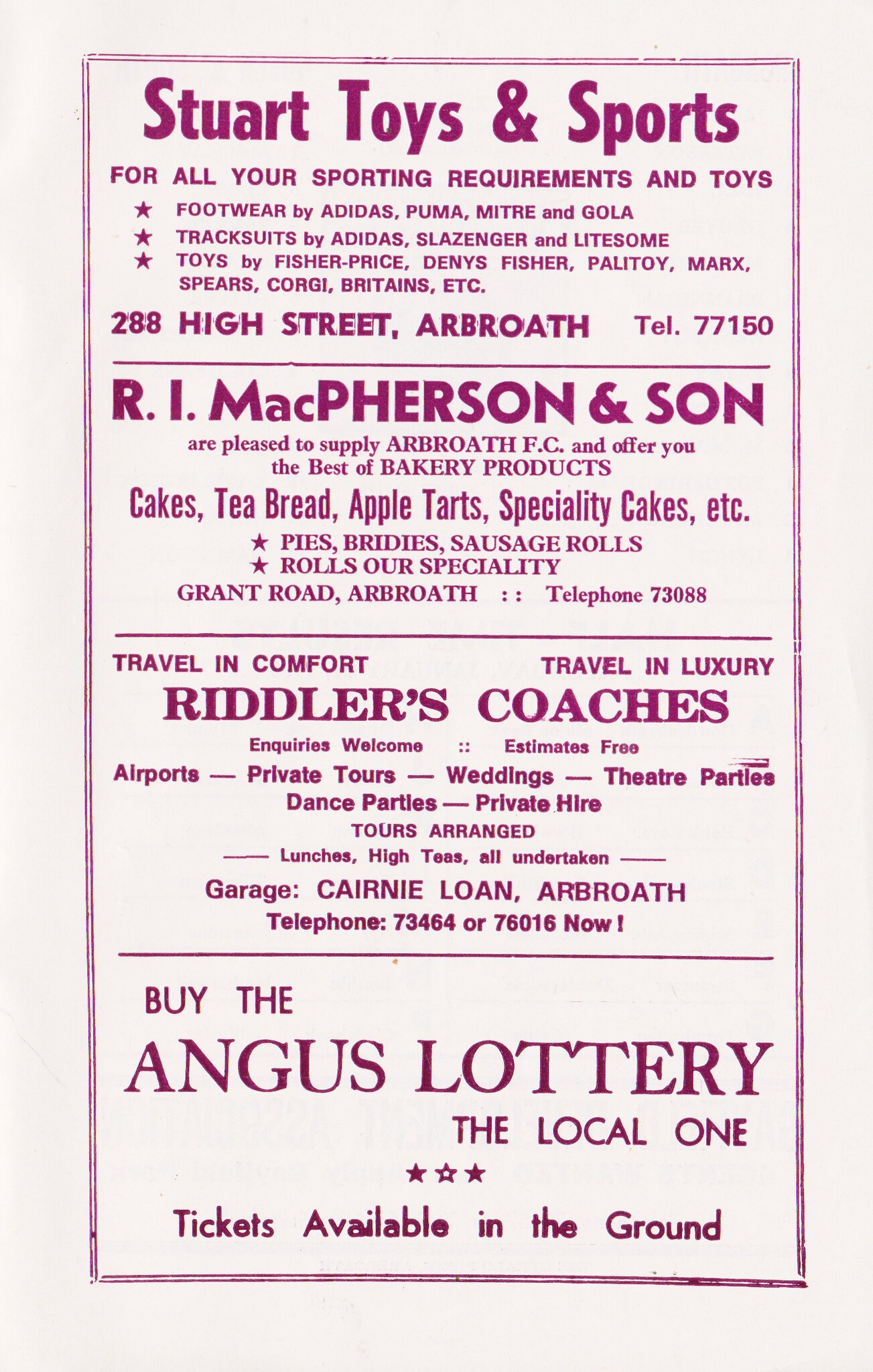This image is a vintage commercial sign featuring a series of advertisements on a white background with black text. At the top, it prominently showcases "Stuart Toys and Sports," emphasizing "For all your sporting requirements and toys," and provides their address at 288 High Street, Arbroath, and the telephone number 77150. Below this, there are three stars followed by a list of products they offer.

Beneath this, the second advertisement is for R.I. McPherson and Son, who proudly supply Arbroath FC and offer a variety of bakery products. Their address is on Grant Road, Arbroath, and their contact details are also mentioned.

The third advertisement promotes Riddler's Coaches, highlighting "Travel in Comfort, Travel in Luxury," and listing their services. The address for Riddler's Coaches is Kearney Loan, Arbroath, with additional contact information provided.

At the bottom, there is an ad for the Angus Lottery, the local lottery, with a note stating that tickets are available on the ground.